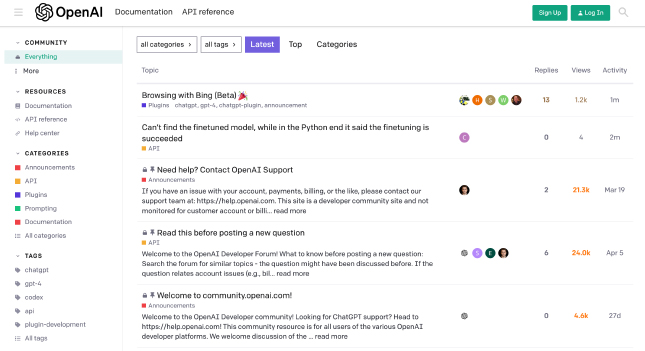A well-organized user interface for the OpenAI documentation and API reference page is displayed on a clean white background. 

- In the top left corner, the words "OpenAI Documentation API Reference" are prominently displayed.
- The top right corner features two green buttons for "Sign Up" and "Login," accompanied by a magnifying glass icon for the search functionality.
- Below the header, a comprehensive menu is situated on the left side, listing various options such as Community, Everything, More, Resources, Documentation, API Reference, Help Center, Categories, and Tags. Subcategories include Announcement, API, Plug-in, Prompting, Documentation, All Categories, Tags, ChatGPT, GPT-4, Codecs, API, Plug-in Development, and AI Tags.
- To the right of the menu, a section labeled "Browsing with Bing Beta" is visible. 
- Below this, a message indicates an issue: "Can't find a fine-tune model." However, in a Python context, it notes that "Fine-tuning has succeeded."
- Additional support information is accessible through a prompt that says "Need help? Contact OpenAI Support," followed by a notice advising, "Read this before posting a new question". 
- A welcoming message at the bottom of the interface reads, "Welcome to community.openai.com."